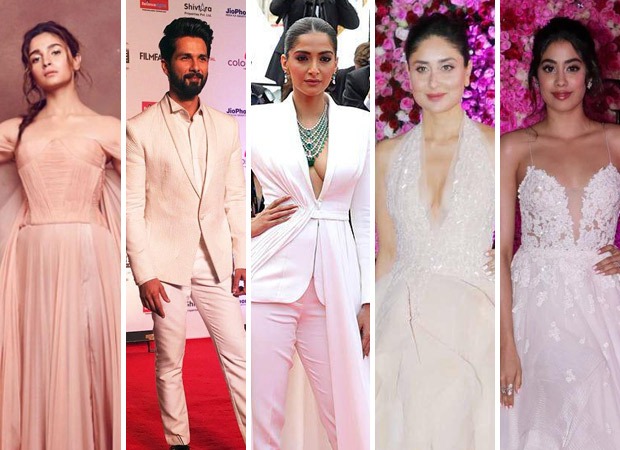This image is a composite split into five vertical panes, each showcasing an individual on a distinctive background, likely from a high-profile red carpet event. The five people positioned left to right include four women and one man, all seemingly Bollywood celebrities due to their ornate attire and features. Each person has black hair and is dressed in white, contributing to a cohesive and elegant visual theme.

In the first panel, a woman is seen in a pale peach-colored dress against a tan background. Her loose, flowing hair cascades over her right shoulder. Next to her, the second panel features a man standing on a red carpet, backed by a wall filled with sponsor logos. He sports a white suit coat, an open-neck white shirt, and white pants. He has black hair, along with a beard and mustache.

The center panel showcases a striking woman in a white tailored pantsuit with a deep neckline, accented by a turquoise geometric necklace. Her sleek, middle-parted hair is pulled back tightly, highlighting her dangling earrings. The background behind her is dark, making her outfit pop.

The fourth panel depicts a woman in a frilly, white halter dress with a bit of sparkle. Her background is a gradient of pink and purple. Her hair is styled intricately on top of her head. The final panel reveals a woman in a strapless, lacy dress reminiscent of a bridal gown. She stands with one hand on her hip, her loose hair styled with tendrils hanging elegantly on the right.